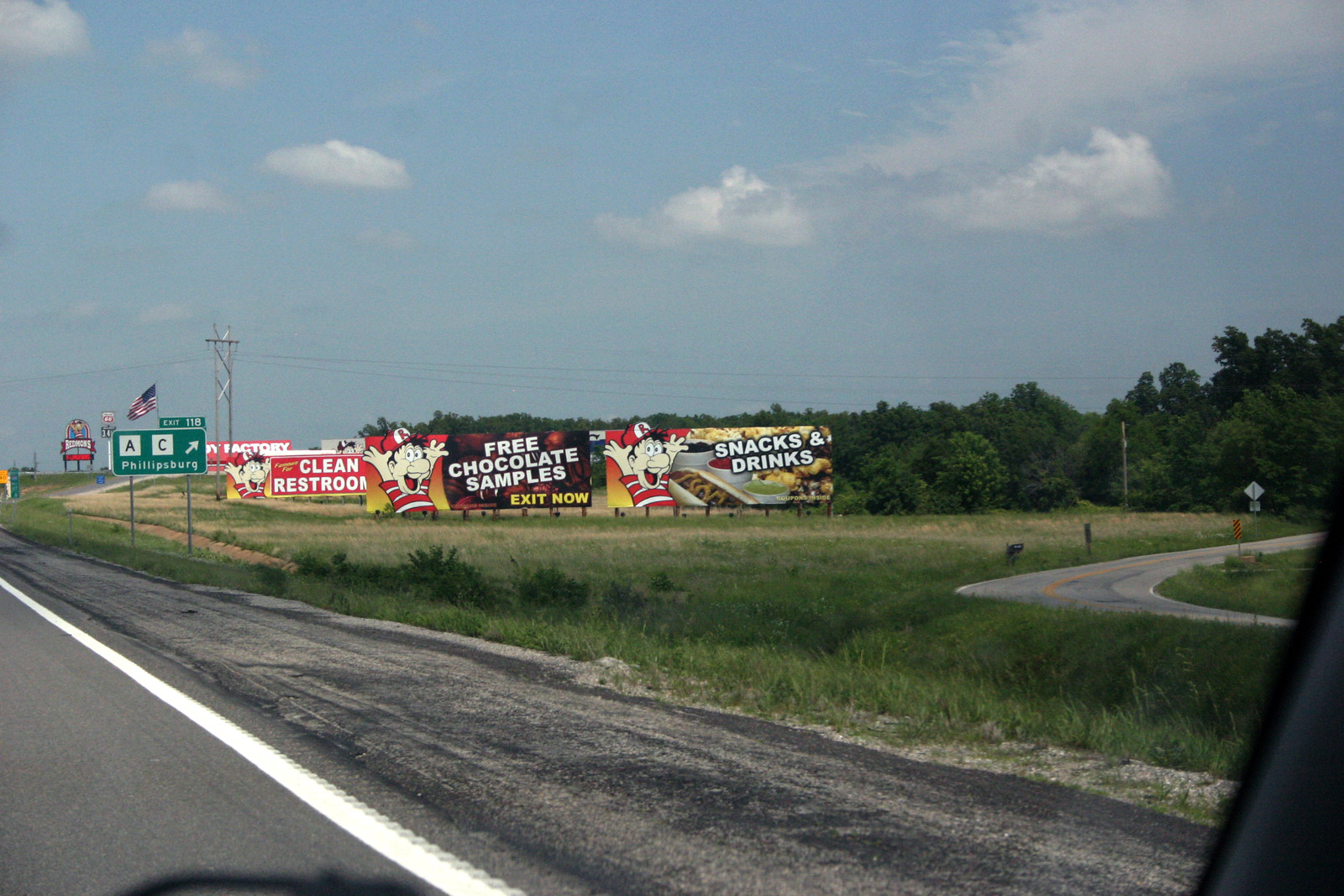The image captures the perspective from within a moving car on the highway, with the windshield edge visible in the lower right corner. A beautiful blue sky with a few scattered gray clouds forms the backdrop, while a dense forest of tall green trees and an expansive grassy field flank the right side of the road. The highway itself is gray, bordered by a long white line and a gravelly black shoulder.

Prominently featured are three yellow and orange billboards clustered together promoting a rest stop. Each billboard showcases a cheerful cartoon boy with his hands up, smiling broadly. The first billboard advertises "Snacks and Drinks," displaying a hot dog image. The next one entices travelers with "Free Chocolate Samples, Exit Now," accompanied by various chocolate images. The final billboard promises "Clean Restrooms," continuing the appealing theme. 

Additionally, there is a green highway directional sign guiding drivers, with sections labeled "A" and "C" and an arrow pointing to the right towards a town starting with the letter "P." The scene includes another road curving into the photo, adding to the sense of motion and anticipation on the journey.